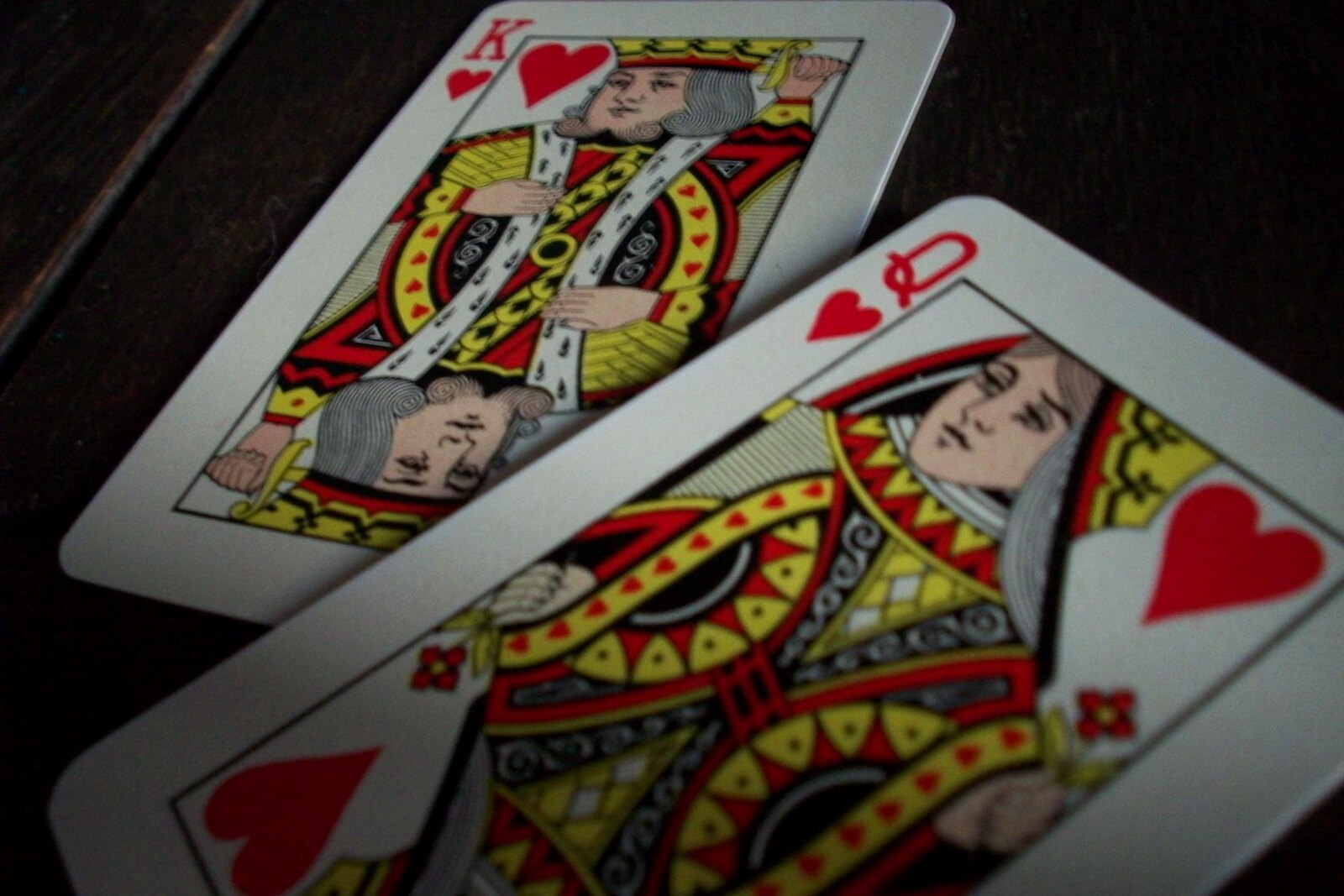This is a close-up photograph of two playing cards, the King of Hearts and the Queen of Hearts, set against a solid black background. The cards, positioned prominently in the frame, are oriented face-up, showcasing their intricate designs. The King of Hearts card is positioned slightly in the background, revealing the king's vivid illustration: he is depicted with a yellow crown, adorned in a yellow-beasted outfit, holding his left hand near his head and his right hand close to his chest. The details of the king's attire include a mix of red and black elements, adding to the regal appearance. Both the upright and inverted images of the king on the card are identical. Overlaying the King of Hearts card at the bottom left corner is the Queen of Hearts card, which slightly occludes the king's bottom right corner. The Queen of Hearts captivates with her elegance, wearing a crown of red, yellow, and black and displaying flowing brown hair. Her attire is a striking combination of red, yellow, black, and white. The prominent 'Q' and heart symbols are also in red, matching the vibrant palette of the cards. Together, these two classic cards create a visually engaging composition against the stark contrast of the black background.